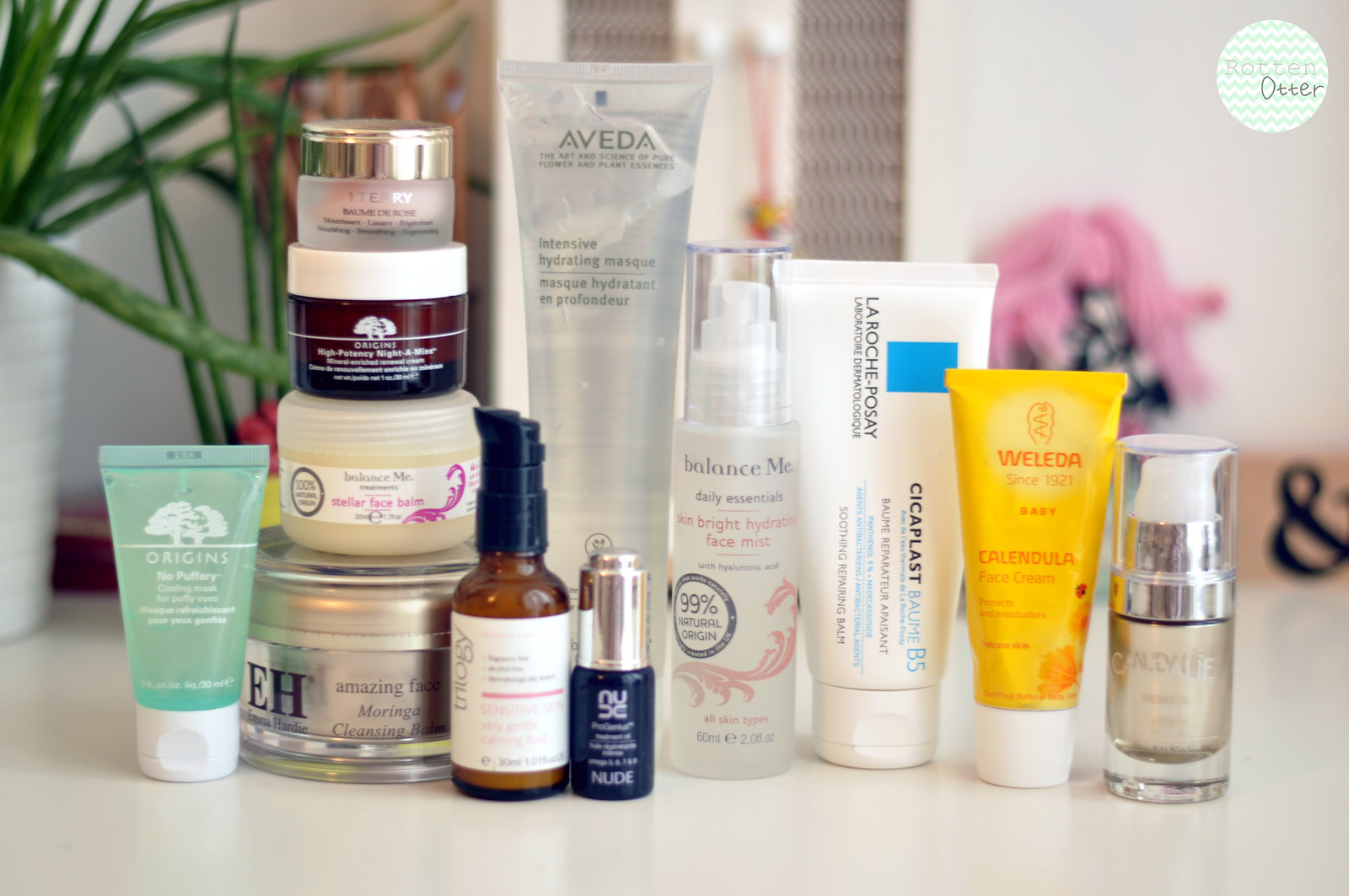The professionally taken photograph features an array of meticulously arranged makeup and skincare products, likely intended for an advertisement. In the top right corner, a logo reading "Rotten Otter" is visible, indicating the brand behind the products. The items are displayed on a table, each positioned to highlight their labels clearly. 

From left to right, the lineup includes:

1. **Origins Cooling Mask for Puffy Eyes**: A small, green bottle designed to soothe and reduce puffiness around the eyes.
2. **Emma Hardie Amazing Face Moringa Cleansing Balm**: A round container at the bottom of a stack.
3. **Balance Me Stellar Face Balm**: Stacked on top of the Emma Hardie container, known for its rich, hydrating properties.
4. **High Potency Night-A-Mins Mineral-Enriched Renewal Cream**: Positioned above the Balance Me balm, aiding in nighttime skin renewal.
5. **The Balm Balm Rose**: The topmost item in the stack, a nourishing balm for various skincare needs.
6. **Trilogy Spray Bottle**: Slightly blurred but identifiable, suggesting a hydrating or setting spray.
7. **Nude Skincare Bottle**: A small bottle providing targeted skincare benefits.
8. **Aveda Intensive Hydrating Mask**: A large bottle in the background, aimed at deeply hydrating the skin.
9. **Skin Bright Hydrating Face Mist**: Another spray bottle to the right of the Aveda product, likely for refreshing and brightening the skin.
10. **La Roche-Posay Balm**: Known for its dermatological benefits, this balm is next in line.
11. **Weleda Face Cream**: Positioned to the right, offering natural and nourishing skincare.
12. **Another Bottle Starting with “C”**: The final product in the lineup, partially obscured, adding an element of mystery to the collection.

The overall composition suggests a sophisticated and diverse selection of skincare essentials, beautifully captured to emphasize their unique features and branding.